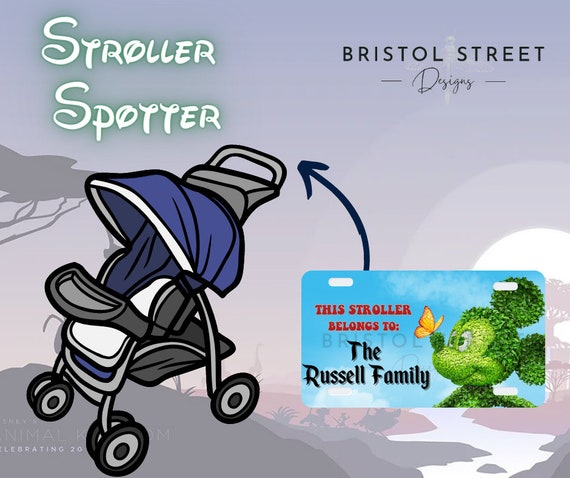The image is a detailed digital illustration advertising the "StrollerSpotter" product by Bristol Street Designs. In the bottom left corner, a large blue stroller with black wheels and a black safety strap is prominently displayed. The stroller is accompanied by a tag in the bottom right corner that reads, "This stroller belongs to the Russell family," featuring an illustration of Mickey Mouse with a butterfly on its nose, suggesting a whimsical Disney theme. The background showcases a gray and white scene reminiscent of Disney's Animal Kingdom, celebrating its 20th anniversary. Additionally, the "StrollerSpotter" name is styled in green Disney font above the stroller. The top right corner of the image features the Bristol Street Designs logo in black and white.